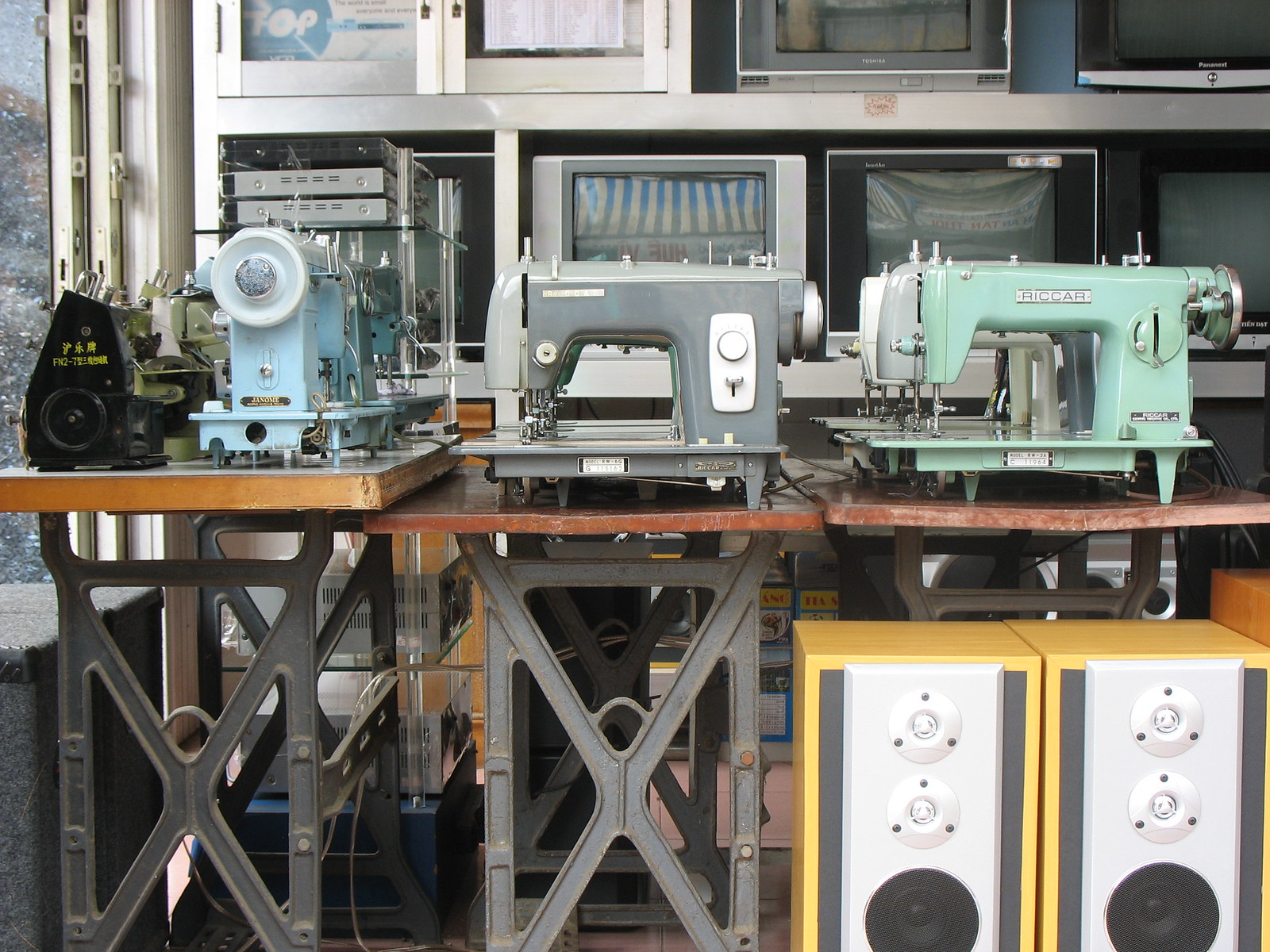This detailed photograph appears to depict a potential retail storage area or an antique store. In the foreground, a series of tables with wooden tops and metal legs featuring X-shaped support beams host an assortment of vintage sewing machines. The sewing machines are diverse in color, including blue, green, gray, and white. Notably, one of the green-covered machines is branded "Ricker." Below these tables, two vertically-oriented speakers with yellow outer casings and white panels sit side by side; each speaker features a dark gray circle near the bottom and two smaller white circles above it. In the background, metal shelves support several small, older television sets, reminiscent of the models common in the late 20th century—these are not modern LCD TVs but rather the bulkier, heavier versions with tinier screens. To the left, a window filters light into the room, and adjacent panels suggest the window can be closed off. Overall, the room exudes a vintage charm, showcasing a variety of older mechanical and electronic devices.